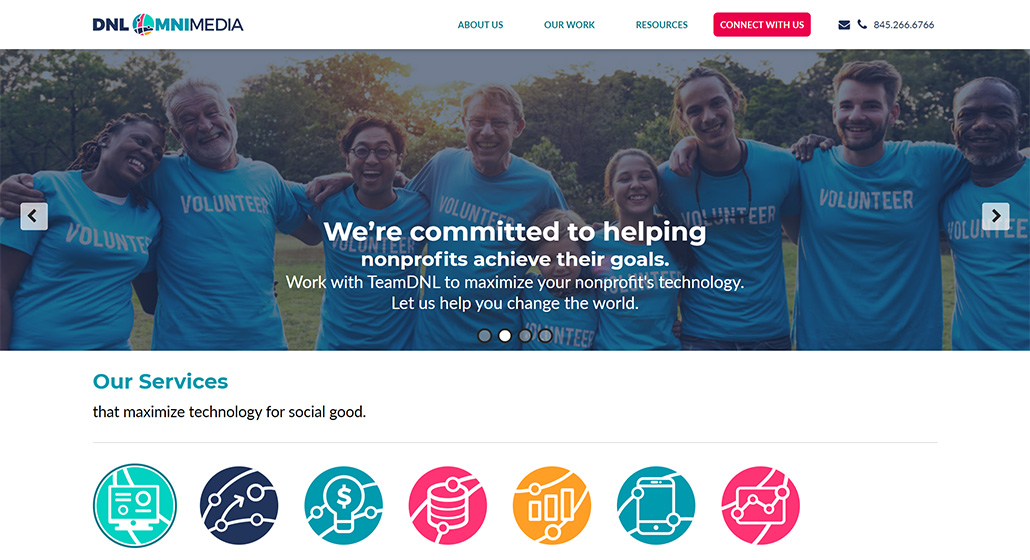This detailed caption describes a screenshot from a website, specifically showcasing an organization dedicated to aiding nonprofits through technology. 

In the upper left corner of the image, the logo "DNL MNI Media" is prominently displayed. The website's navigation bar features several clickable options: 'About Us,' 'Our Work,' 'Resources,' 'Connect With Us,' and a contact number, 845-266-6766.

Central to the screenshot is a vibrant photo depicting a group of smiling individuals, all clad in blue shirts emblazoned with the word "Volunteer." Accompanying the image is a motivational message: "We're committed to helping nonprofits achieve their goals. Work with Team DNL to maximize your nonprofit's technology. Let us help you change the world."

Below this message, a subheading reads "Our services that maximize technology for social good," followed by a series of seven icons, each housed within small circles. These icons symbolize various services offered:
1. A computer, likely indicating IT support or digital solutions.
2. A network chart, signifying connectivity or organizational networking.
3. A light bulb with a dollar sign, perhaps representing financial innovation or cost-effective ideas.
4. A stack of coins, denoting financial management or fundraising.
5. A graph, possibly indicative of data analysis or performance tracking.
6. A phone, likely highlighting customer support or communication services.
7. Another chart or graph, suggesting data visualization or strategic planning.

This screenshot effectively conveys the organization’s mission to empower nonprofits by leveraging technology to create meaningful social impact.